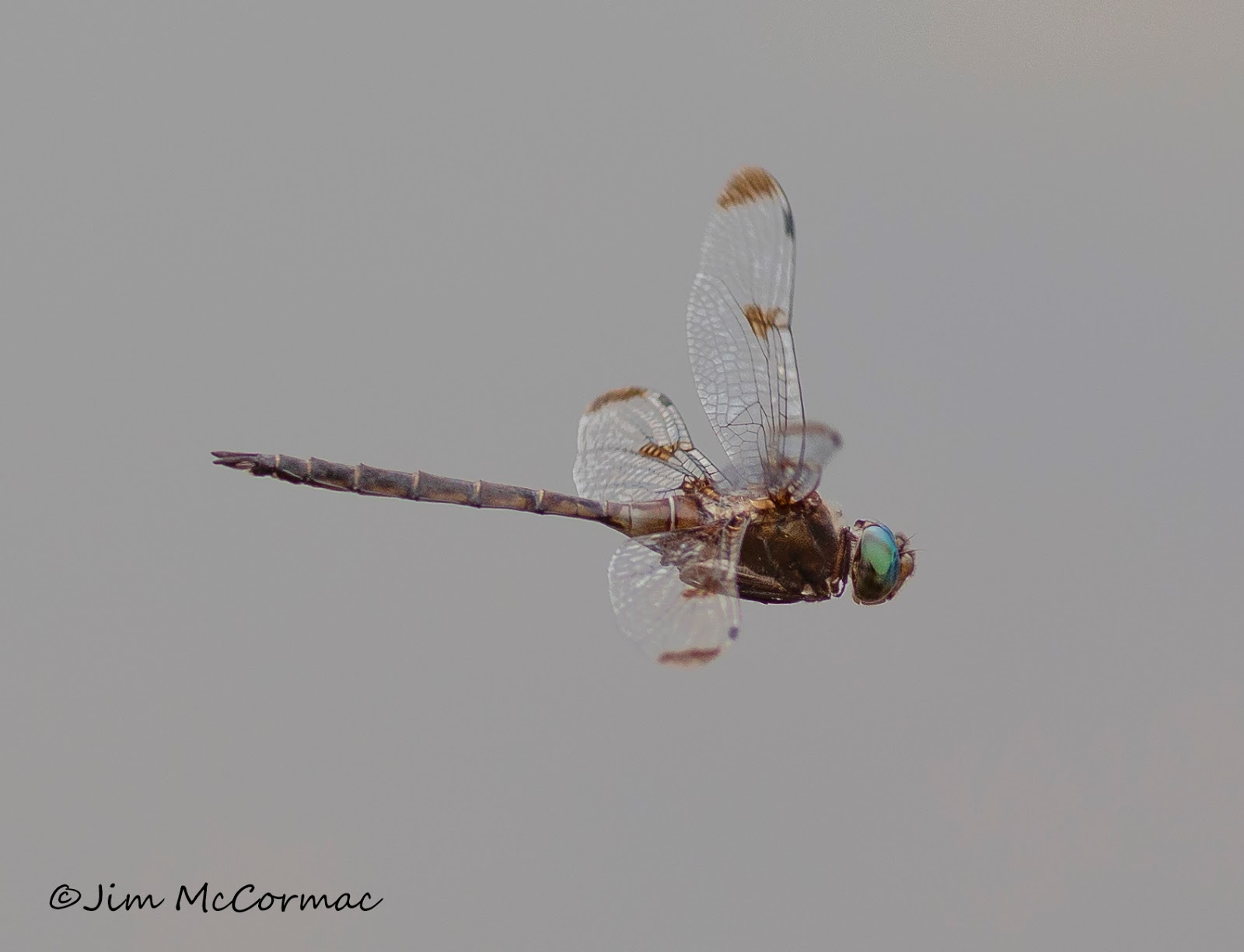A detailed, close-up photograph of a dragonfly in mid-flight against a grayish-white background. The dragonfly is oriented from left to right, with its head, a striking bluish-green color, prominently in the foreground. Its sizable, shiny eyes reflect the light, creating an almost emerald-like appearance. The dragonfly's body is elongated and segmented, showcasing a mix of dark and light brown hues, and the thorax appears dark and metallic. Its four translucent wings, which seem almost frozen in motion, exhibit delicate brown spots and edges. The wings, sprouting from the middle of its body, add to the intricate detailing of the photograph. The image is signed with a copyright symbol and the name "Jim McCormick" in the lower left corner, attributing the masterful capture to the photographer.